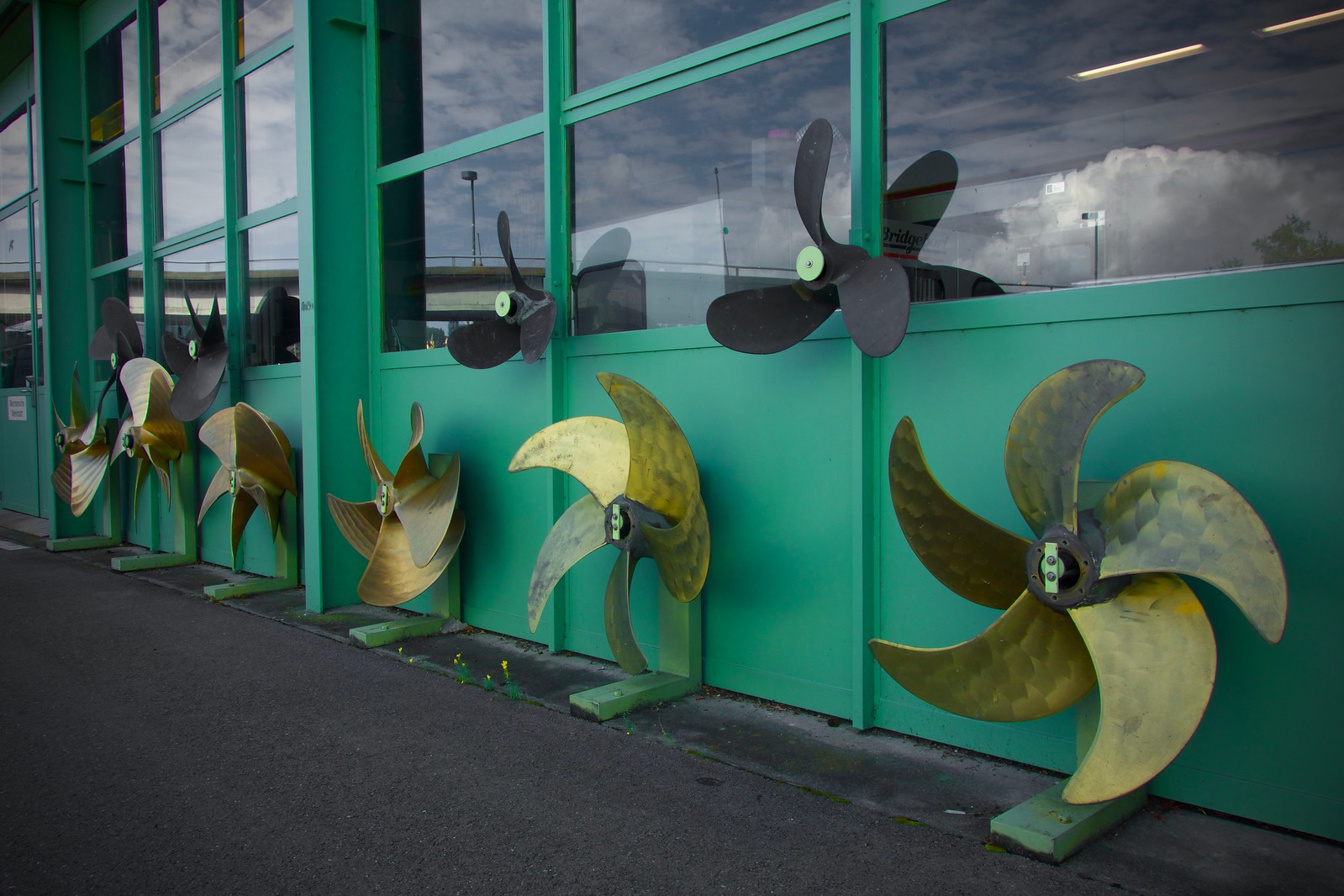The image showcases a green building featuring numerous windows and an array of unique, hand-created fan or propeller structures attached along its exterior. The wall of the building is light green and glass panels are visible above. There are approximately ten fan models, some bolted to the wall and others positioned on the ground. These fans or propellers vary in design and number of blades; for example, one has five blades while another has four, and two fans just above have three blades each. The fans have curved blades, differing in color and pattern with some appearing black and others bronze. These diverse structures create an intricate aesthetic display against the green backdrop of the building. In the bottom left corner, part of the street—which is black in color—can also be seen. It remains unclear whether these are functional devices or simply artistic sculptures.